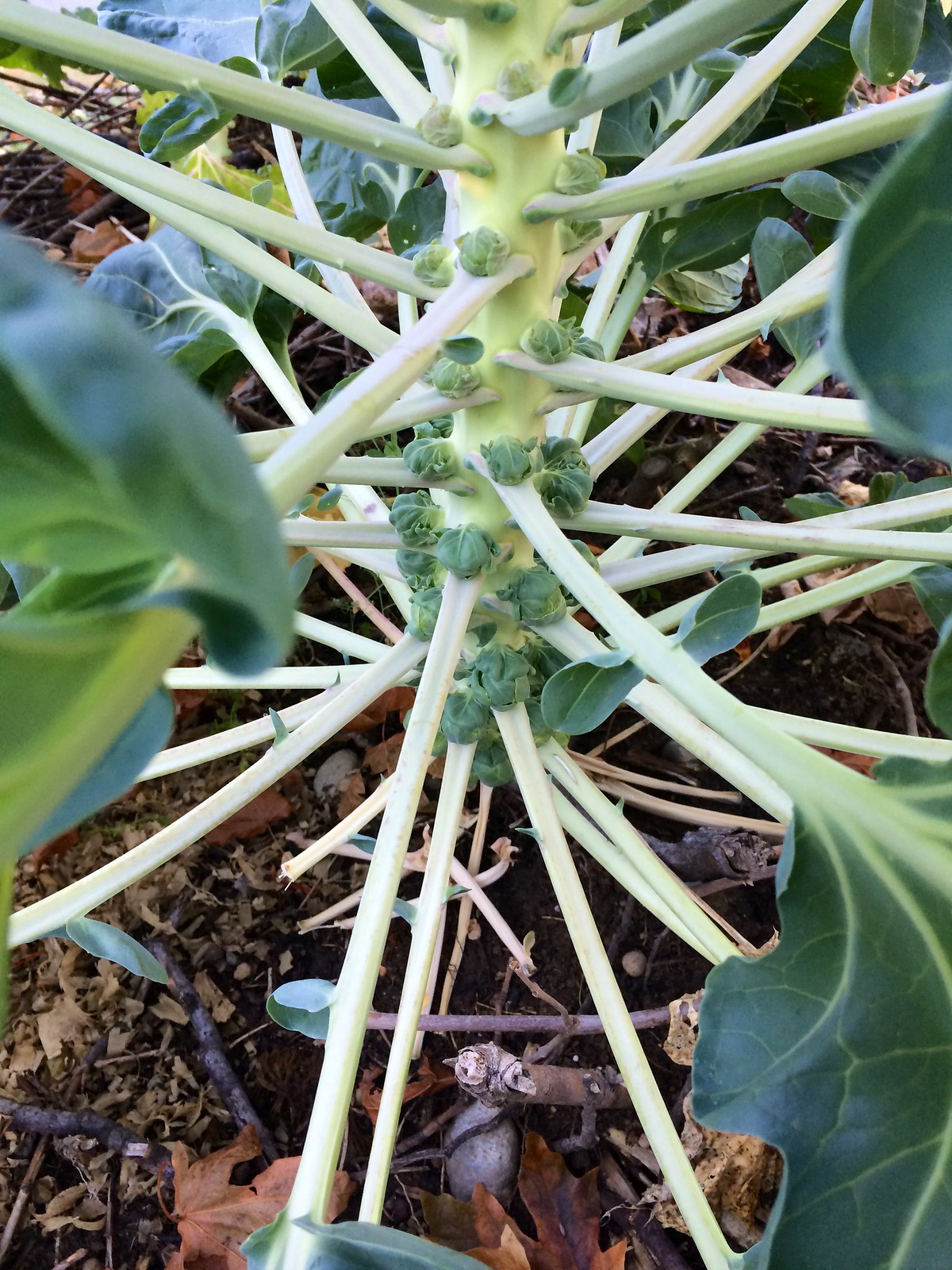This high-quality, close-up color photograph captures the detailed richness of a Brussels sprout plant from an almost 45-degree downward angle. The central stem of the plant, a light green hue, ascends vertically with numerous lighter green to nearly white horizontal stems spiraling outward. At the ends of these horizontal stems, large, dark green leaves spread out, their lighter green veins creating a striking contrast. Nestled around the circumference of the main stem are small, dark green buds, which will eventually develop into Brussels sprouts. The plant is embedded in earth, with the surrounding ground dotted with twigs, sticks, brown and orange autumn leaves, and a few pebbles.